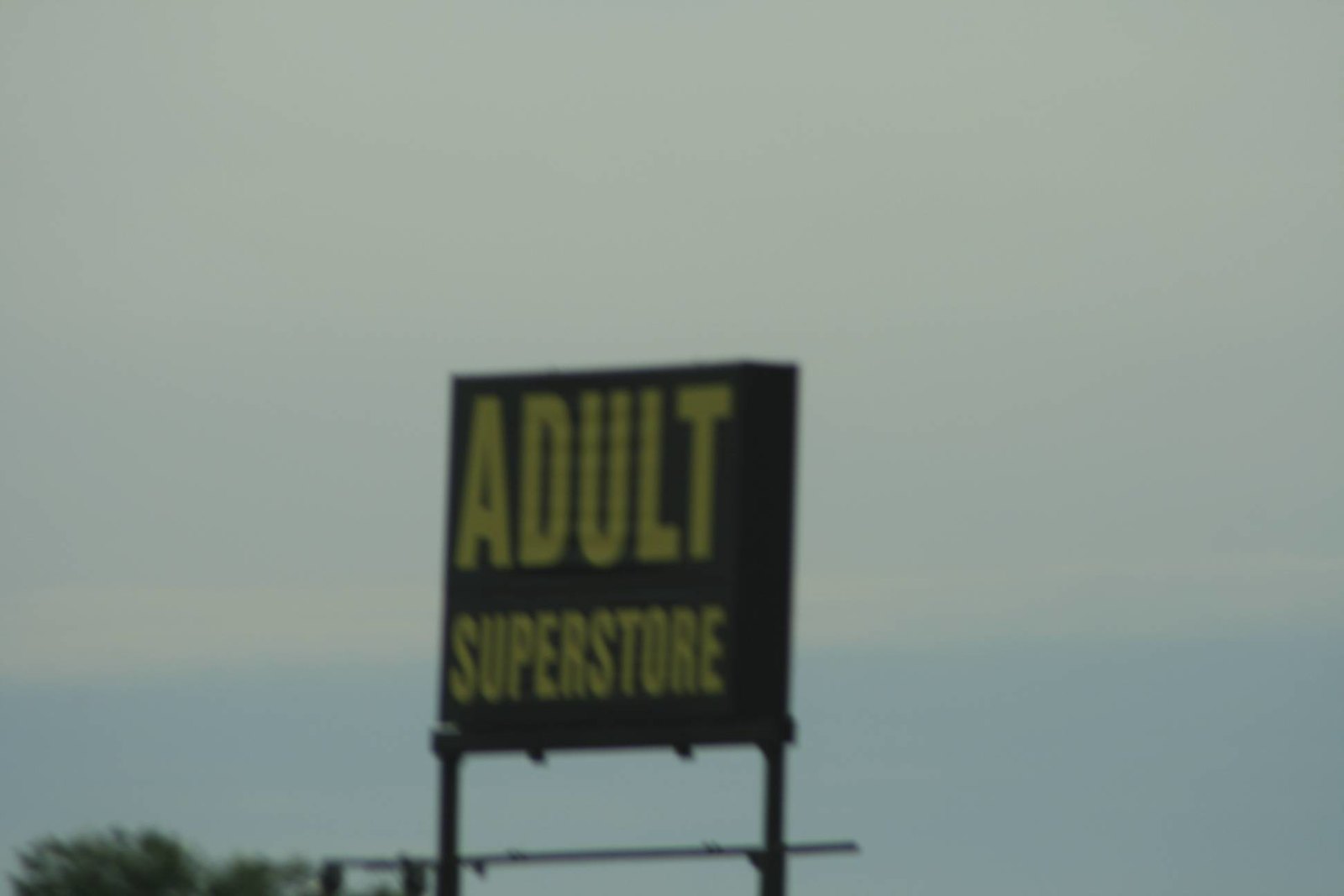The image captures a large, square-shaped sign standing prominently against a mostly white, overcast sky with faint blue shading at the bottom. The sign, resembling a billboard, is black with bold yellow lettering that reads "ADULT" in very large letters and "SUPERSTORE" in smaller letters beneath. It is supported by two black poles on either side, with a third horizontal pole running perpendicular beneath it. Additionally, the sign appears to have a lighting assembly, possibly for illuminating the text at night, although this feature is somewhat indistinct due to the blurry nature of the photo. The lower left corner of the image shows a fuzzy, greenish portion of a tree protruding, adding a touch of organic contrast to the stark sign. The entire scene is captured at an upward angle, giving the impression of looking up towards the sign from below.